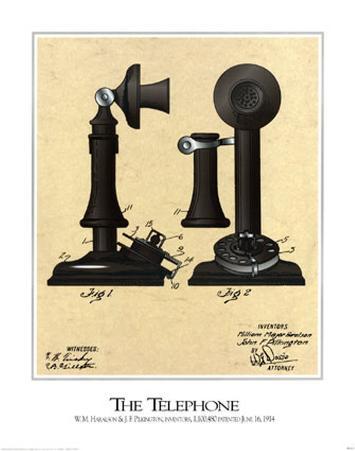This is an illustrated drawing of a very early telephone, possibly from the early 1900s. The main image is surrounded by a square, gray border and features two labeled figures: figure 1 on the left, showing a side view of the telephone, and figure 2 on the right, displaying a front view. The telephone itself is black, with a dial turner on the base—a type where you insert your finger, rotate it, and it cranks back after release. The device has a separate earpiece that you would hold to your ear, while speaking into a fixed mouthpiece. Beneath the image, in large capital letters, is the caption "THE TELEPHONE." There is additional text underneath this caption, though it is too small and blurry to read clearly. The detailed markings in figures 1 and 2 demonstrate the different parts and functions of the telephone, and a signature appears in the bottom right corner.